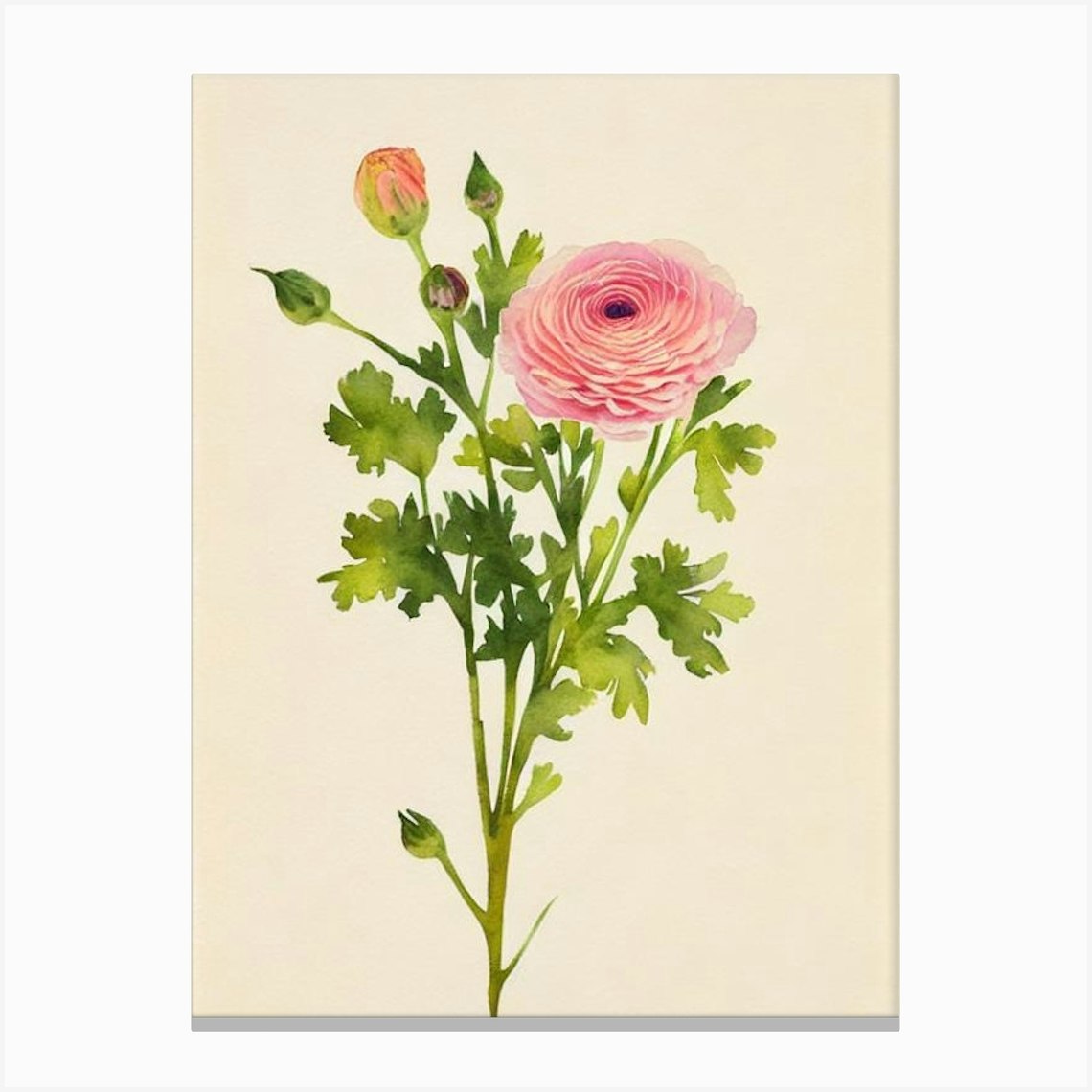The image is a detailed watercolour painting of a rose and several rose buds on a beige rectangular canvas, oriented vertically. Centered in the painting is a green stem with varying shades of green leaves and a solitary thorn near the bottom. At the top right of the stem is a fully open, light pink rose with lush, layered petals, resembling a peony. To the left of the open rose, there are four rose buds in different stages of bloom. The lowest bud is entirely green, the next higher is green with hints of purple, the one at the mid-level is green with streaks of purple, and the highest partially open bud has pink petals with red streaks emerging from a green base. The arrangement of the flowers and leaves highlights a play of light, creating a dynamic depth and texture in the composition.